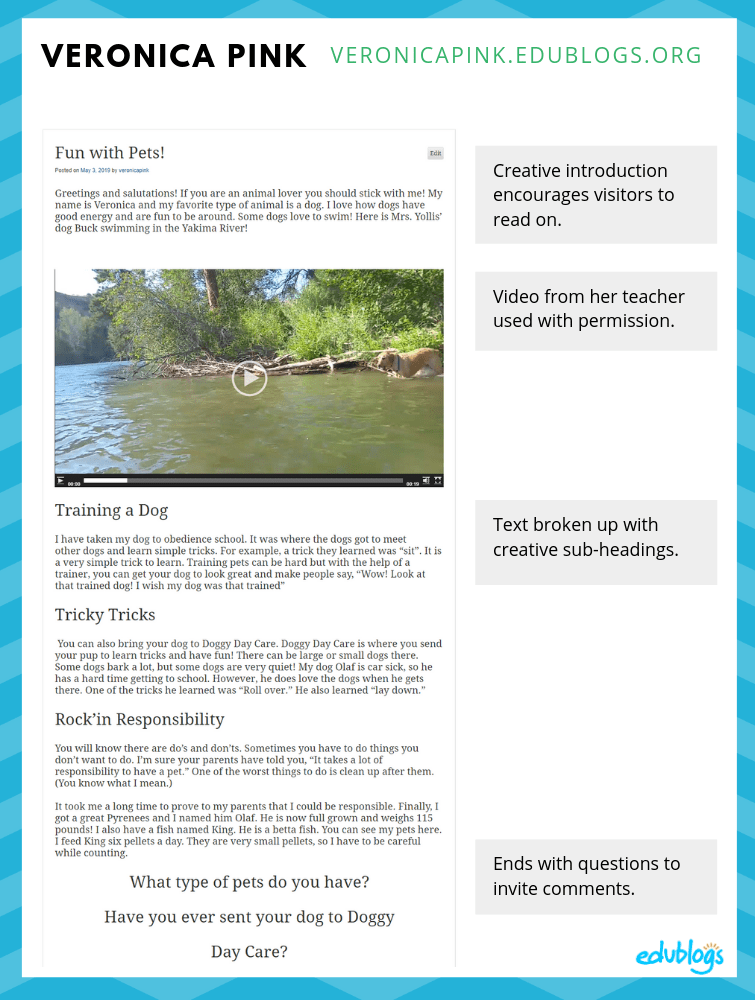This image features a vibrant banner with the text "Veronica Pink Black" prominently displayed. The banner is divided into several sections, with the top right featuring the website URL "veronicapink.edublogs.org" written in green letters. Adjacent to this, on the far right, there is a green box labeled "Fun with Pets." Below this label is a post with detailed explanations connected to the third section.

On the left side of the banner, a creative introduction encourages visitors to delve deeper into the content. Accompanying the introduction is a video thumbnail showing a dog by a serene lake. To the right of the thumbnail, a gray box contains the caption "Video from her teacher used with permission."

Below the video section, the content is divided into three neatly organized sections: 

1. "Training a Dog"
2. "Tricky Tricks"
3. "Rockin' Responsibility"

Each section is clearly separated with creative subheadings, and the text is broken up for easy reading. At the bottom of the banner, a prompt encourages reader engagement with the phrase "End with quick questions to invite comments."